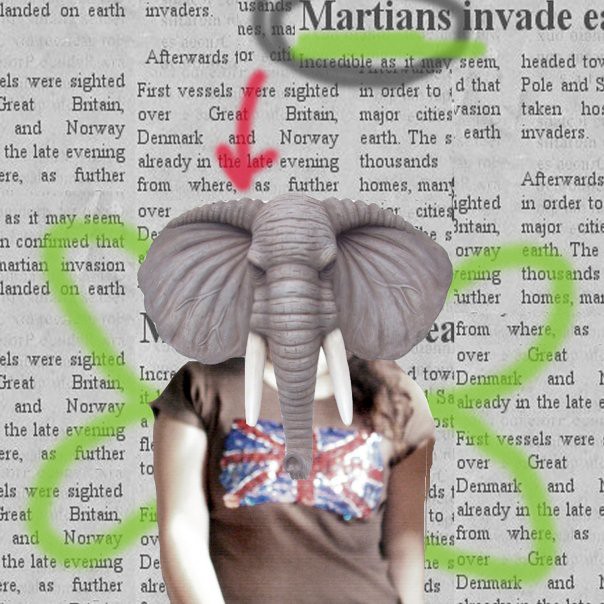This digital art project features a surreal collage that combines photography with digital illustration. The background consists of overlapping newspaper clippings, making the text largely unreadable except for the prominent headline "Martians Invade." The word "Martians" is emphasized with a grey circle and a green underline, and a red arrow points downward from the headline. At the center of the image, a striking digital illustration of an elephant's head is placed on a human body. The figure, which appears to be a white woman, is wearing a brown t-shirt adorned with a glittery British flag, featuring the red and white stripes against a blue background. Surrounding this central figure, green butterfly wings are digitally drawn, further enhancing the fantastical nature of the artwork.